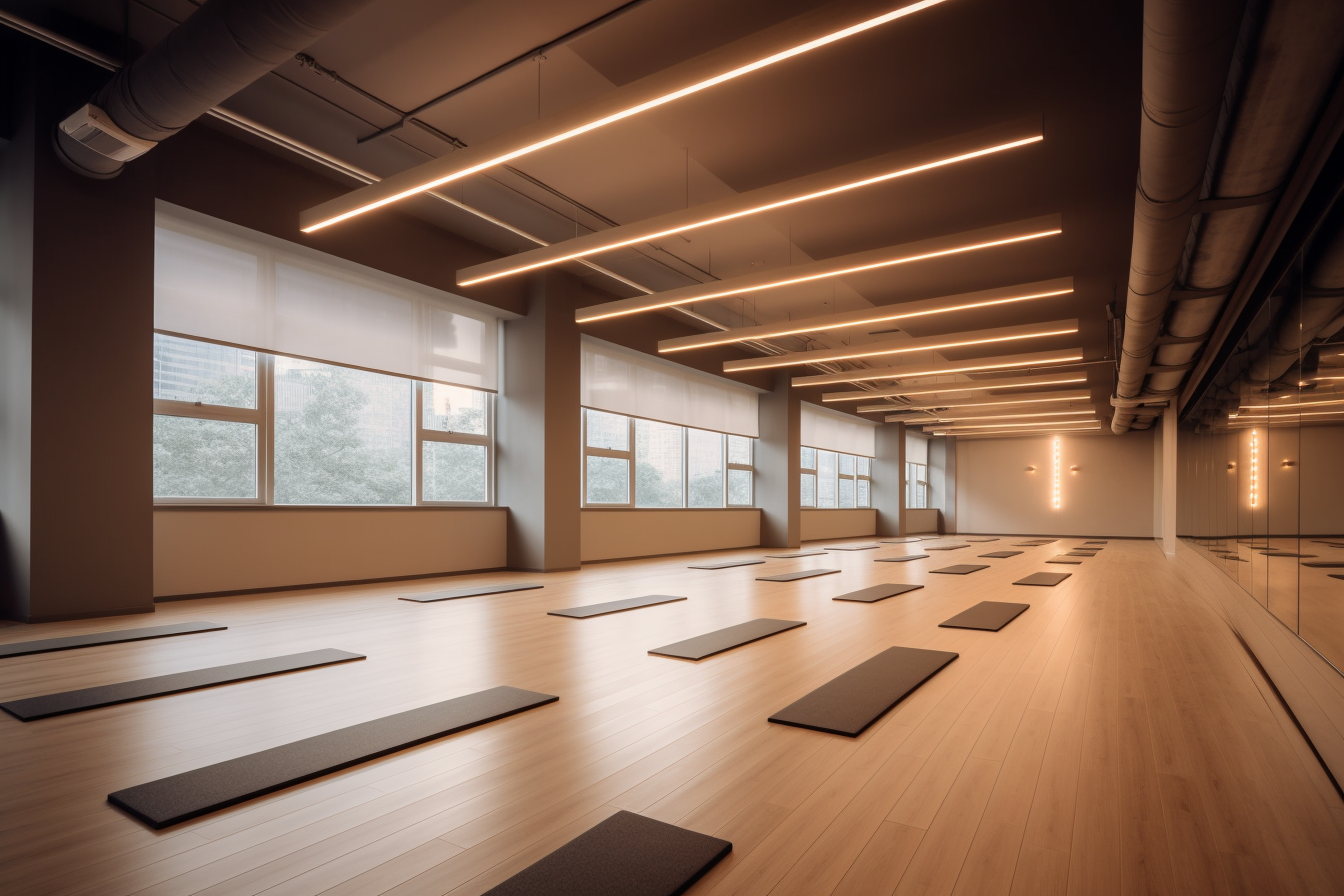This image is a detailed color photograph of the interior of a yoga studio, likely an architectural rendition. The space is a large, long, and narrow room, approximately 80 feet in length, emphasizing its spaciousness. The flooring is light-colored wood, resembling a gym floor, and is adorned with yoga mats, although inconsistencies in their shapes suggest some may be digitally rendered.

The right wall is entirely covered with mirrors, reflecting the expanse of the room, while the left side features a series of large windows comprising three segments each, flanked by window blinds currently pulled up. These windows allow daylight to flood in, enhancing the bright ambiance of the space. Above, long strips of lighting run horizontally across the ceiling and down the walls, extending from the windows to the mirrored wall. The ceiling, a medium brown color, also houses visible air vents and pipes, adding to the functional yet stylish design of the studio.

At the far end of the room, a light bar feature adds a focal point, and the walls are painted a light tan color, contributing to the calm and serene atmosphere ideal for yoga practice.